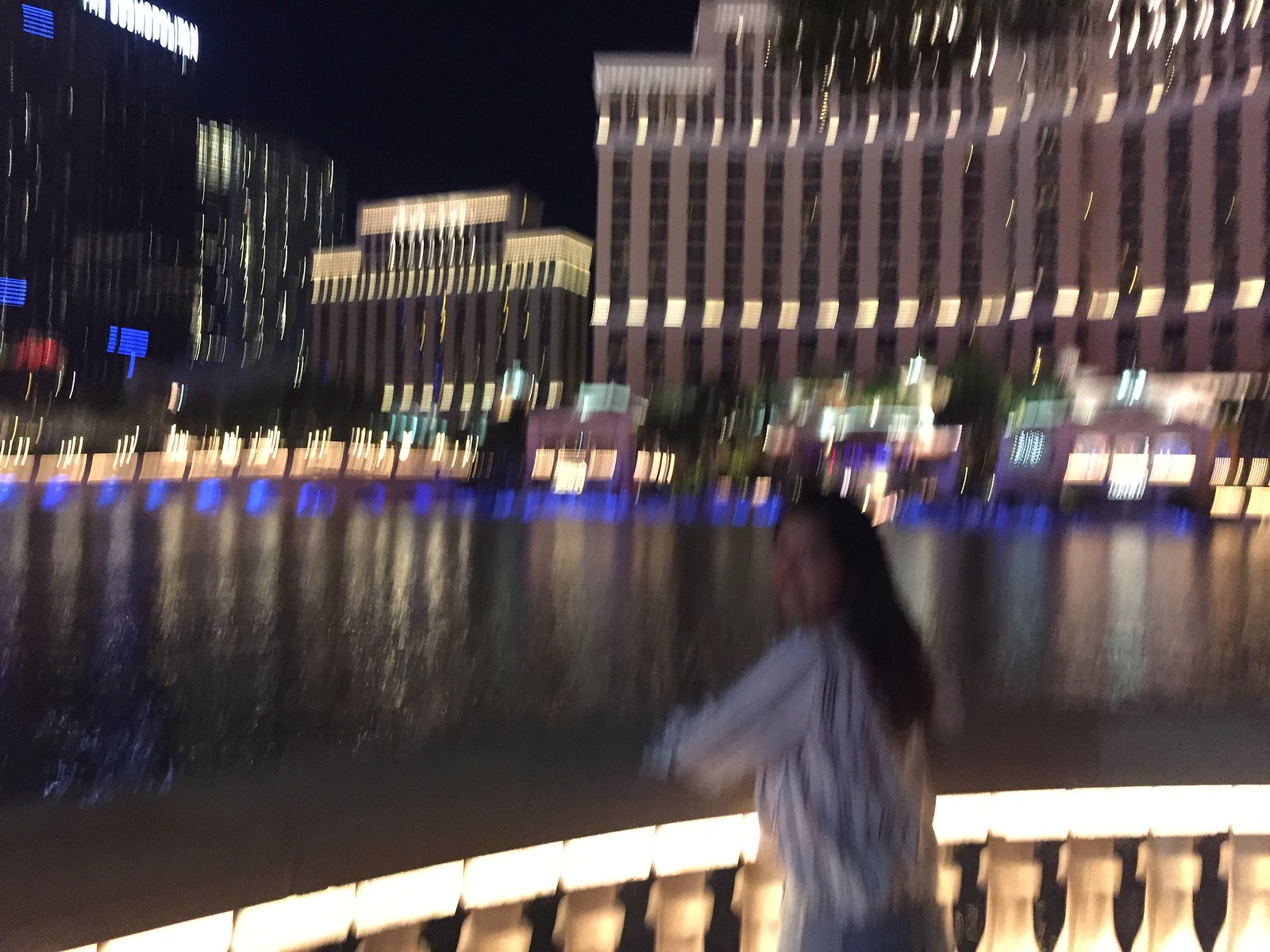Despite the image being blurry, it captures a striking scene: A woman stands at a curved banister overlooking what appears to be a lake, distinctly placed in the middle of a cityscape. The water body, possibly a lake given its dark hue, contrasts with the urban surroundings. To the right, there is an extensive brick-colored hotel characterized by its multitude of vertical columns and alternating window patterns, countable at around seventeen. Adjacent but slightly set back is a shorter building of a similar design, though its roof is of a lighter shade. To the top left of the image, a business named "Power Eyes" is discernible, though the text is somewhat obscured due to the image's clarity issues. The scene provides a unique juxtaposition of natural and architectural beauty within an urban setting.